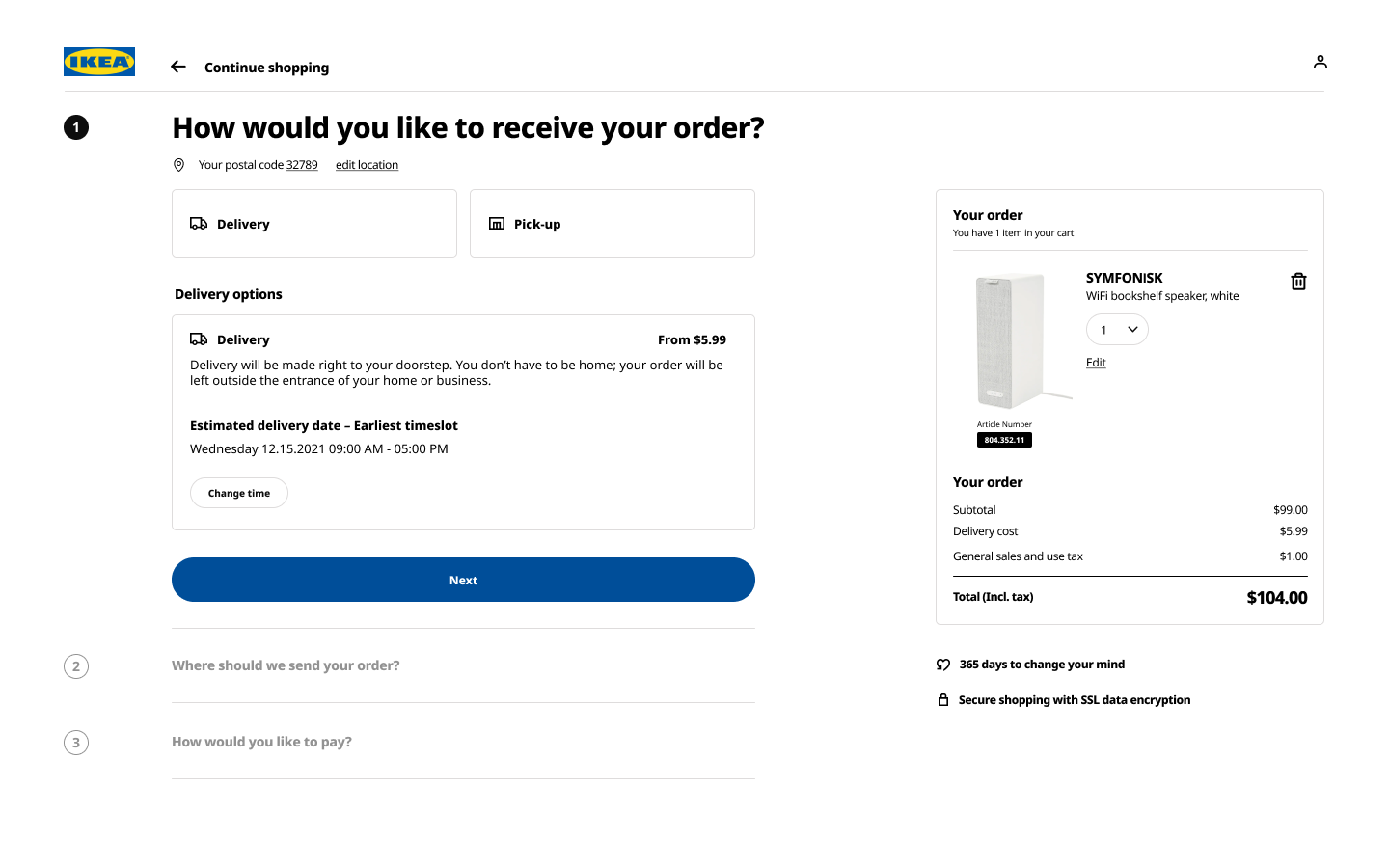This image captures a detailed view of the IKEA website's checkout page, meticulously organized into three main sections.

At the very top, there's a distinctive header featuring the IKEA brand logo, an intuitive back arrow for returning to the shopping experience, and a "Continue Shopping" option.  

The central section, spanning the majority of the page, is bifurcated vertically. On the left side, it prominently asks, "How would you like to receive your order?" This section includes an editable postal code field and presents two options via buttons: delivery or pickup. Below, a rectangular box titled "Delivery Options" details the delivery price of $5.99, alongside an estimated delivery date. There's an additional button for adjusting the delivery time, complemented by a large blue "Next" button. Further steps outlined underneath pertain to confirming the delivery address ("Where should we send your order?") and payment method selection ("How would you like to pay?").

The right-hand side, extending from top to bottom, summarizes the order details. This segment itemizes the products in the cart, the subtotal, delivery cost, sales tax, and the overall total. The bottom part of this section reassures customers with notes regarding the 365-day return policy and the security of their shopping experience, highlighted by SSL data encryption.